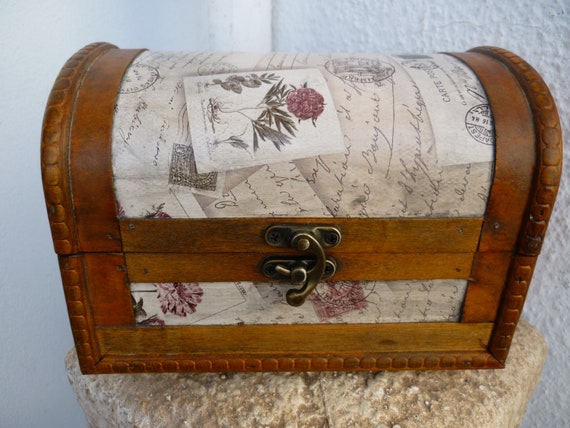The image depicts an old-fashioned, small chest resting on a flat, off-white, slightly bumpy stone or cement pedestal. The chest features a rounded lid that meets a square base, secured by a brass-colored latch that turns to keep the lid closed. The design combines elements of dark brown leather-like material covering the seams and corners, with center panels adorned with printed images of old cursive French text and the words "carte de postale." Accentuating these vintage graphics are pictures of pink and reddish flowers, possibly chrysanthemums, adding an elegant touch to the nostalgic aesthetic. The background consists of a highly textured, rough white wall, reminiscent of a popcorn ceiling.